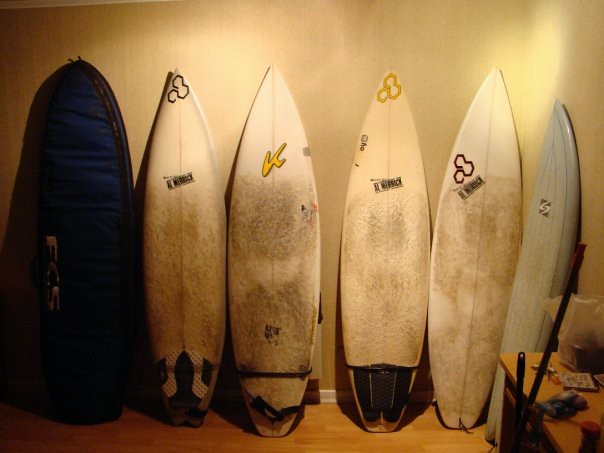In this color photograph, six surfboards are neatly lined up against a light yellow, beige, or mustard-colored wall, possibly under artificial lighting that gives the image a yellowish sepia tint. These boards rest on a wooden floor that appears to be light oak in tone. Five of the surfboards are visibly well-used, smudged, and dirty, predominantly off-white in color. They feature various logos, such as a yellow "K," three interlocking circles, and a thunderbolt motif. The surfboard on the far left is encased in a black or dark blue zippered cover, possibly hinting at an additional or empty board inside. To the right of the arrangement, a small workbench or table is partially visible, cluttered with miscellaneous items, adding to the scene's indoor, workshop-like setting.